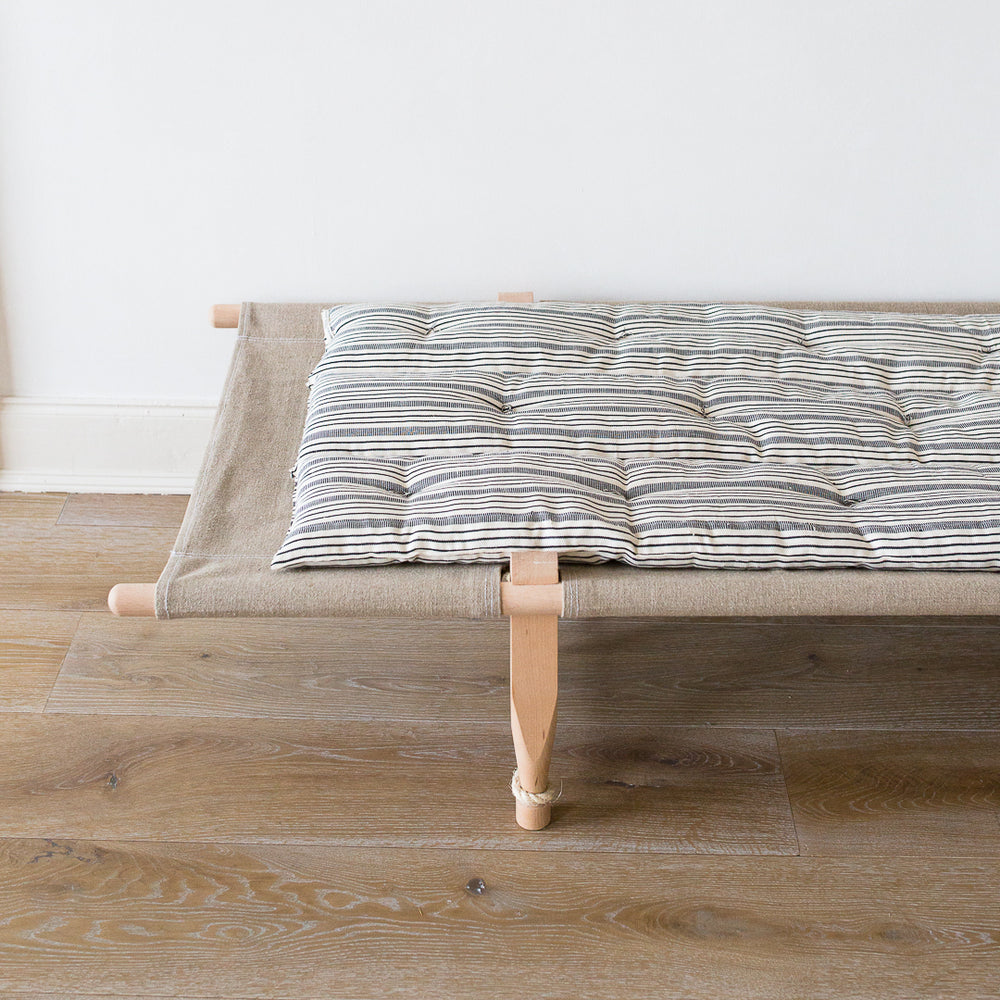This photograph showcases a modest, beige-gray canvas cot set against the backdrop of a pristine white wall and baseboard. The cot's natural light-colored wooden legs extend upward to rounded posts, and a piece of rope is tied around one leg just an inch above the wooden-paneled floor. The cot itself features a stitched canvas fabric in a light brown hue. On top of the canvas surface lies a small quilted cushion, cream-colored and adorned with fine stripes in shades of dark blue and bluish-gray, adding a subtle touch of texture and pattern to the rustic simplicity of the scene.